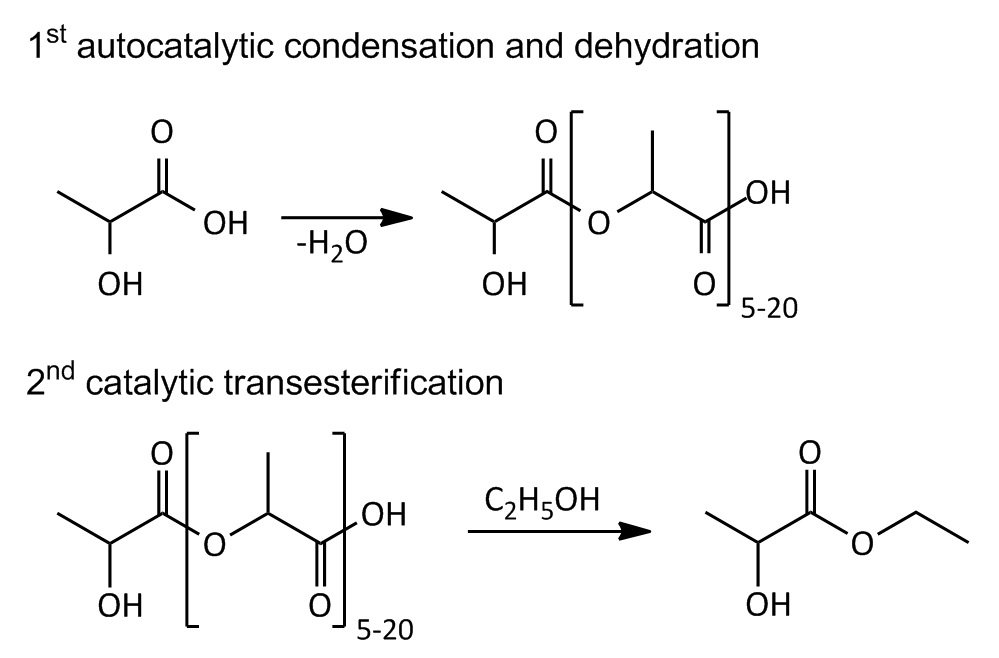This black-and-white image, likely an excerpt from a textbook, provides detailed chemical diagrams illustrating two processes: autocatalytic condensation and dehydration, and catalytic transesterification. At the top, labeled "First Autocatalytic Condensation and Dehydration," the diagram showcases molecular structures featuring elements such as O (oxygen), OH (hydroxyl), and water (H2O). The structures are connected by single and double bonds with arrows indicating the removal of H2O, transforming into a new configuration labeled 5-20, depicting changes in the molecular arrangement.

The bottom section, labeled "Second Catalytic Transesterification," presents a similar style of diagrams. It begins with molecular structures involving O, OH, and the compound C2H5OH. An arrow points to a new structure representing the final product of the transesterification process, again labeled with configurations that include O and OH groups.

The image, devoid of any background color or borders, strictly focuses on these chemical transformations, featuring concise black text and schematic diagrams, making it a precise scientific illustration of the described chemical processes.